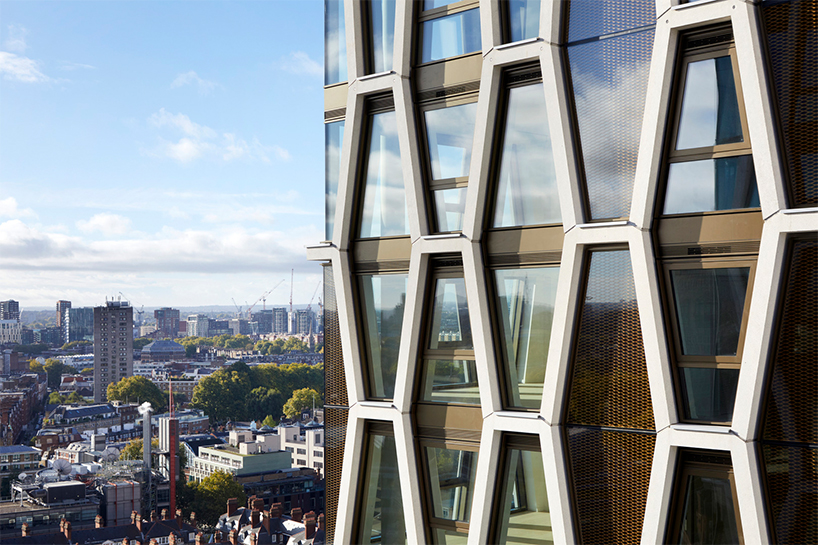The image captures a vibrant urban skyline from a high vantage point, showcasing a striking contrast between a close-up modern skyscraper on the right and a sprawling cityscape in the background. The dominant building to the right features numerous large, coffin-shaped windows split into a top and bottom part, framed by light brown paneling. Its unique design includes a honeycomb-like hex pattern, reminiscent of a beehive, and reflects the surrounding cityscape in its glass facade, with hints of green interiors visible. The background reveals a variety of buildings, ranging from short to towering skyscrapers, some under construction with visible cranes. The lower part of the image is dotted with chimneys and other architectural details, while the upper portion features a stretch of blue sky and white clouds. Far off in the distance, a line of trees is visible, possibly leading to a distant ocean or mountain range, adding depth to the expansive urban scene.